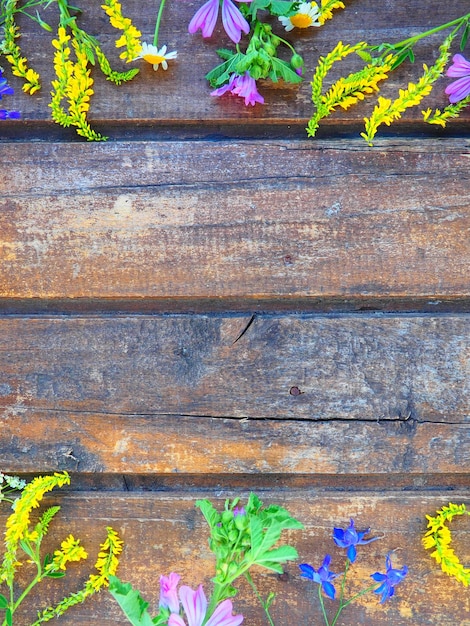The image depicts a weathered wooden surface, likely a porch or deck, seen from above. The wooden planks are aged, showing signs of wear with splits and cracks in various shades of brown, black, orange, and white. Nail points are visible in the planks, adding to the rustic appearance. Strewn across the top and bottom portions of the wooden surface are multiple flowers, not quite mirroring each other but similarly arranged as if scattered. The flowers include bright yellow blooms, light purple petals with green, bushy leaves, small blue flowers with delicate petals, and a white daisy with a yellow center. The origin of the flowers is unclear; they appear to simply lay artistically on the wooden panels, creating a vibrant contrast with the weathered wood background.